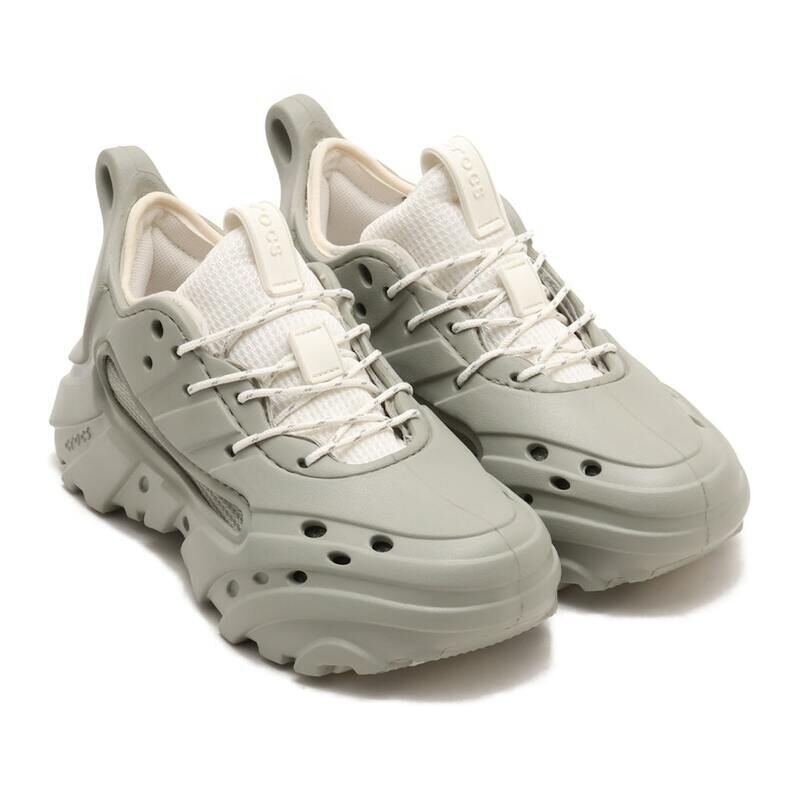The image features a pair of light gray athletic shoes with distinctive Crocs branding. The shoes, which bear a strong resemblance to Crocs in style, are primarily made from silicone-like plastic. They have numerous circular cutouts or ventilation holes along the sides for breathability. The shoes feature white laces and a white lip with the Crocs logo. The interior of each shoe is cushioned and white or off-white. Additionally, there's a heel loop at the back for ease of wearing. The photograph, taken on a white background, highlights the shoes with shadows under the toes, emphasizing their three-dimensional form and construction.